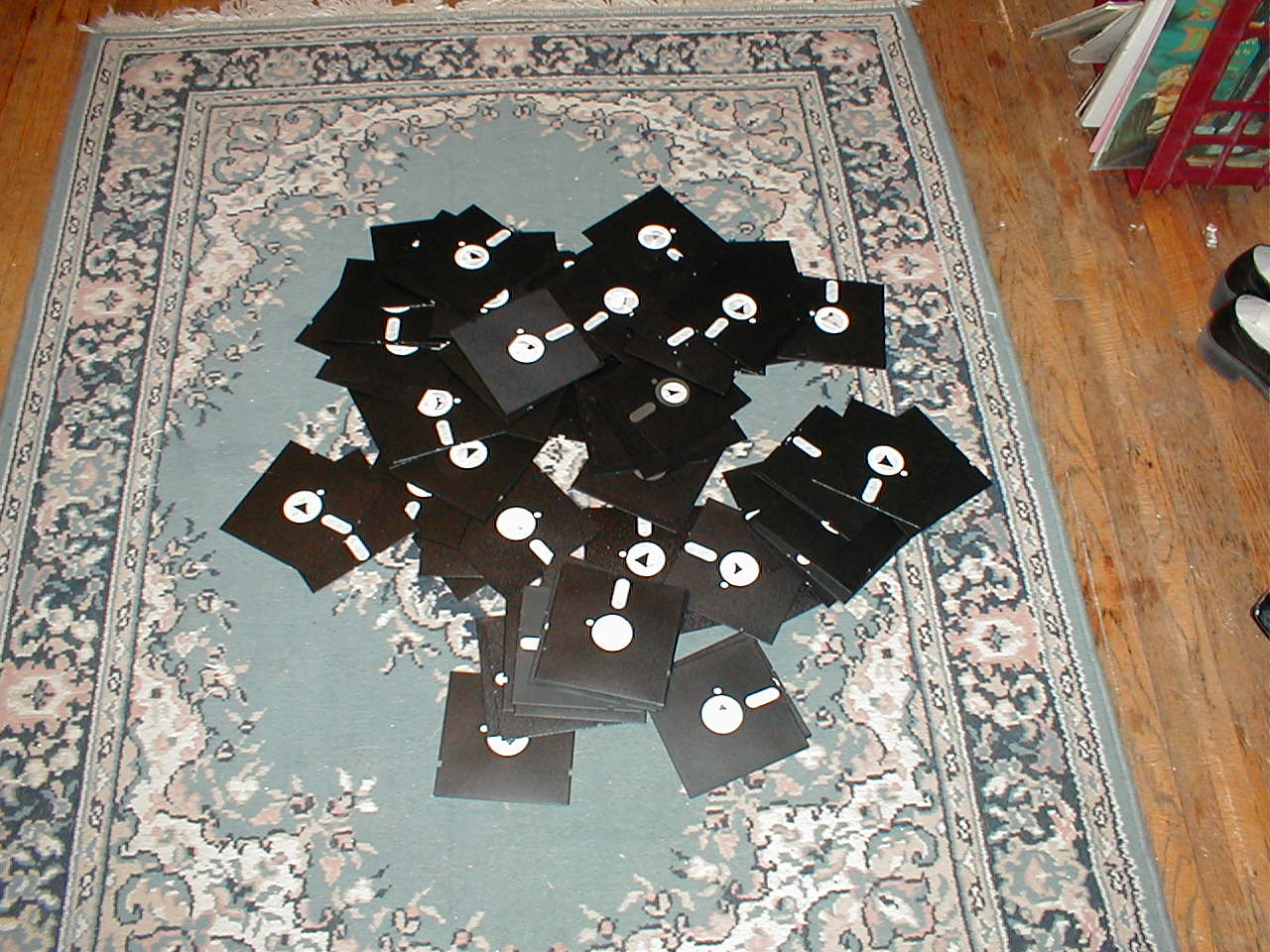This photograph captures an eclectic scene where a disorganized pile of old black floppy disks dominates the center of a richly detailed, vintage blue-gray rug. These very old floppy disks, with white centers and adjacent white labels, are haplessly scattered about, suggesting they were recently dumped from their cases. The rug beneath features an intricate floral and scroll design, with hints of pink interwoven among its mainly teal blue background. This rug, bordered by fine, decorative fringes at its top and bottom, but not at the sides, appears to rest on a mahogany hardwood floor. To the right of the rug and disks, the wooden floor is partially visible, alongside a pair of shoes cut off at the edge of the image. Additionally, a magazine or record stand is seen housing some records and magazines, contributing to the nostalgic mood of the setting.